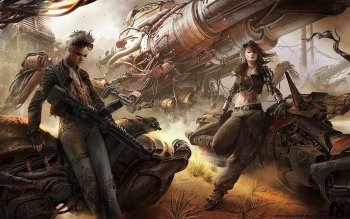This detailed illustration depicts a post-apocalyptic scene featuring two women standing confidently on top of rugged motorcycles. Both women exude a tough, punk vibe, sporting leather jackets, leather tank tops, and cargo pants. The woman on the right has long, flowing brown hair and is dressed in a midriff-bearing top and dark cargo pants cinched with a black belt. She leans against her motorcycle, her stance accentuating her readiness and strength. To her left, the second woman wears jeans and a gray or black blazer, with a large machine gun slung over her shoulder, its barrel pointing downward. The background reveals a massive, destroyed machine, its insides gutted and wires ripped out, hinting at a recent battle or looting. The dark, grim color scheme amplifies the warlike atmosphere, emphasizing the chaotic and perilous world they inhabit.